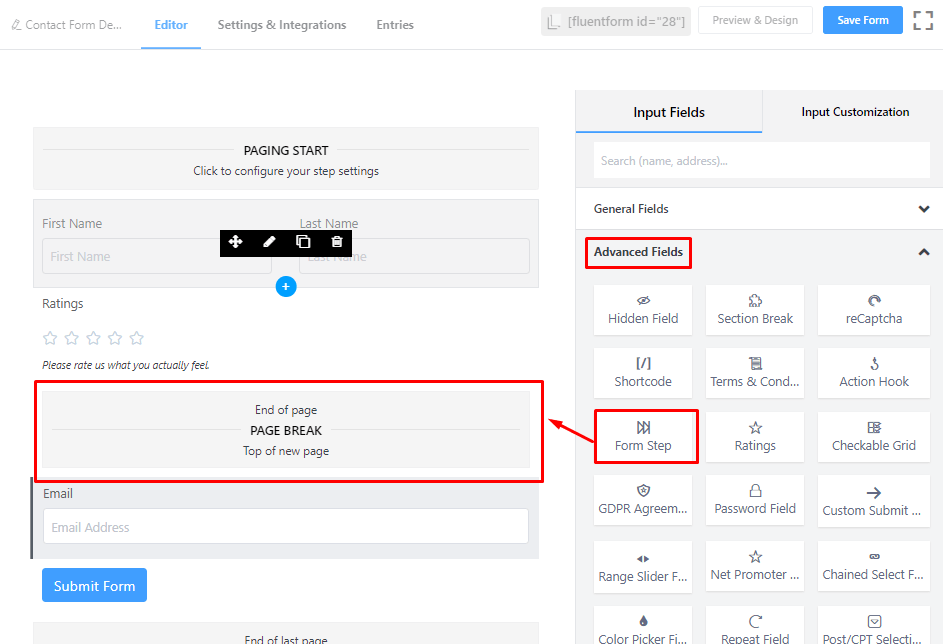In this screenshot of a settings page for a contact form, the top of the page displays the title "Contact Form DE" which is partially cut off. The "Editor" section, highlighted in blue, appears to be the active tab among the options "Settings," "Integrations," and "Entries."

Displayed as "Fluent Form ID = 28," the interface provides options such as "Preview," "Design," and a prominent blue "Save Form" button. Below this, there is a section labeled "Paging Start," with a prompt to "Click to configure your step settings."

The form features input fields for "First Name" and "Last Name," over which a small black tooltip box appears. This box includes icons for editing (a pen), deleting (a trash can), and splitting windows. Below these fields, there is a rating system with five empty stars and the instruction to "Please rate what you actually feel."

A red rectangular box highlights the "End of Page" section, which includes a "Page Break" and an "Top of New Page" label, followed by a field for "Email Address" and a blue "Submit Form" button.

On the right side of the page, there are sections labeled "Input Fields" and "Input Customization." The "Advanced Fields" section is highlighted in red and includes various field options such as "Hidden Field," "Section Break," "ReCAPTCHA," "Short Code," "Terms and Conditions," "Action Hook," "Form Step," "Ratings," "Quick Checkable Grid," "GDPR Agreement," "Password Field," "Custom Submit," "Range Slider," "Net Promoter," "Change Select," "Color Picker," "Repeat Field," "Post CPT," with "Form Step" specifically surrounded by a red box indicating its selection.